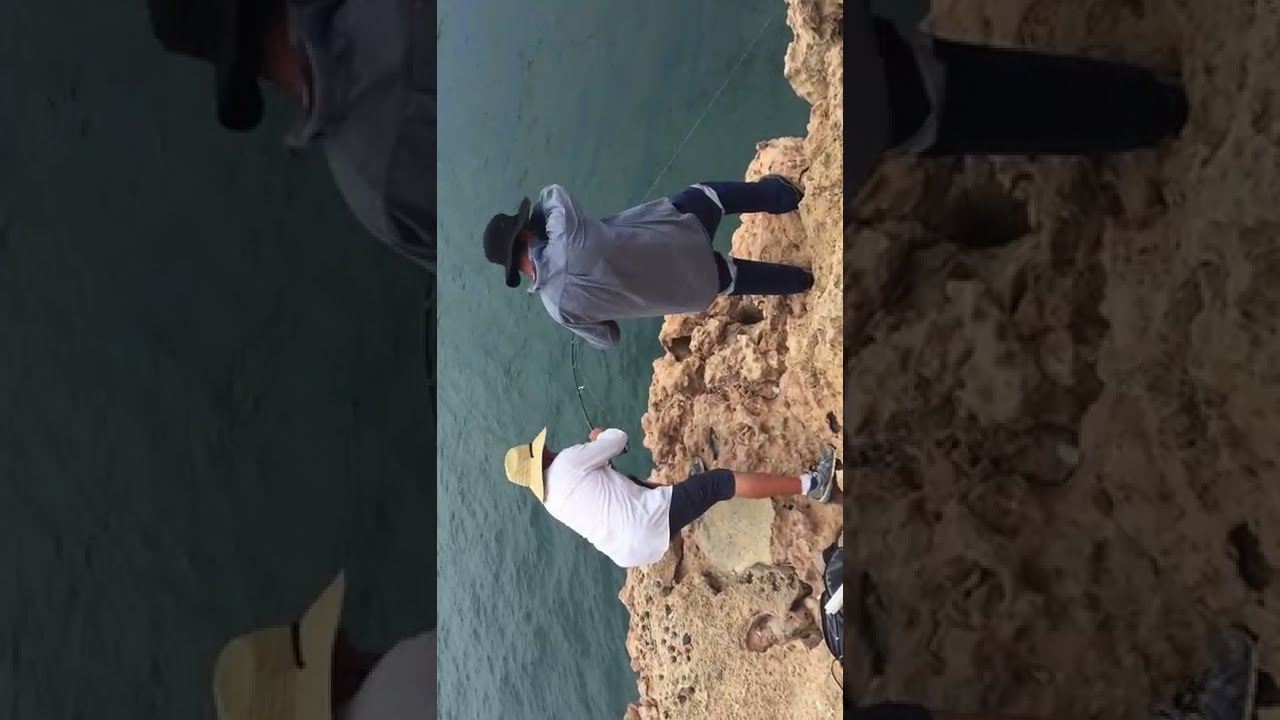In this photograph, which has been rotated counterclockwise, we see two men fishing on a rocky shoreline beside a large body of blue ocean water. The scene appears to be set outdoors on a bright, clear day. The men are central to the image, each equipped with fishing poles dipped into the water.

The man positioned on what is now the bottom of the image (originally the left side) is wearing a beige straw hat, a white long-sleeve shirt, three-quarter shorts, and sneakers. He stands on the rocky surface, appearing to struggle with his fishing pole, perhaps indicating he has caught something. 

The other man, located on the upper part of the photo (originally the right side), dons a black hat and a long-sleeve collared shirt that is untucked, along with long pants. His posture suggests discomfort, as he has his arms raised and his eyes covered, possibly shielding them from sunlight or debris. 

Together, the men are engrossed in their fishing activity against a backdrop of blue water and light brown-gray rocks, creating a scene rich in natural colors like blue, tan, beige, white, and hints of yellow and silver.